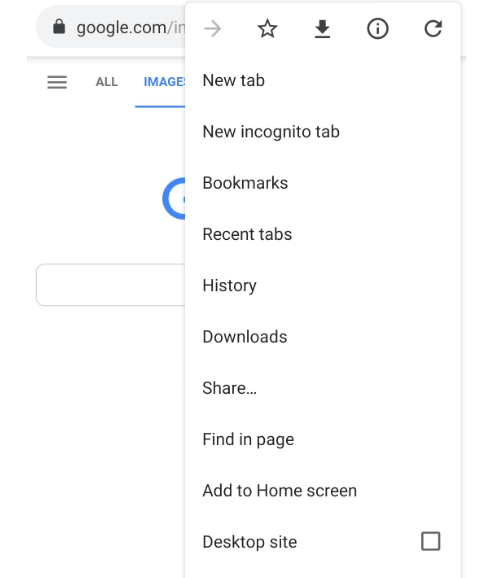### Detailed Caption:
This image is a screenshot of a Google search page. At the very top, the address bar is visible, showing "google.com" as the URL. Directly below the address bar is a standard white background that characterizes the Google search page, although the search box itself is obscured by a pop-up menu that takes center stage in the image.

The pop-up menu has a white background and across the top, a row of icons is aligned horizontally. These icons include an arrow pointing to the right, a star, a download icon, a circle with an eye in it, and a refresh button. Underneath this row of icons is a list of black text options in the following order:

1. New Tab
2. New Incognito Tab
3. Bookmarks
4. Recent Tabs
5. History
6. Downloads
7. Share
8. Find In Page
9. Add to Home Screen
10. Desktop Site

Each text option appears clearly on the white background of the menu. The overall layout of the image suggests that this pop-up menu is likely part of the Google Chrome mobile browser, and it offers various navigational and utility options to the user. The search page in the background is largely obscured by this menu, making it the focal point of the image.